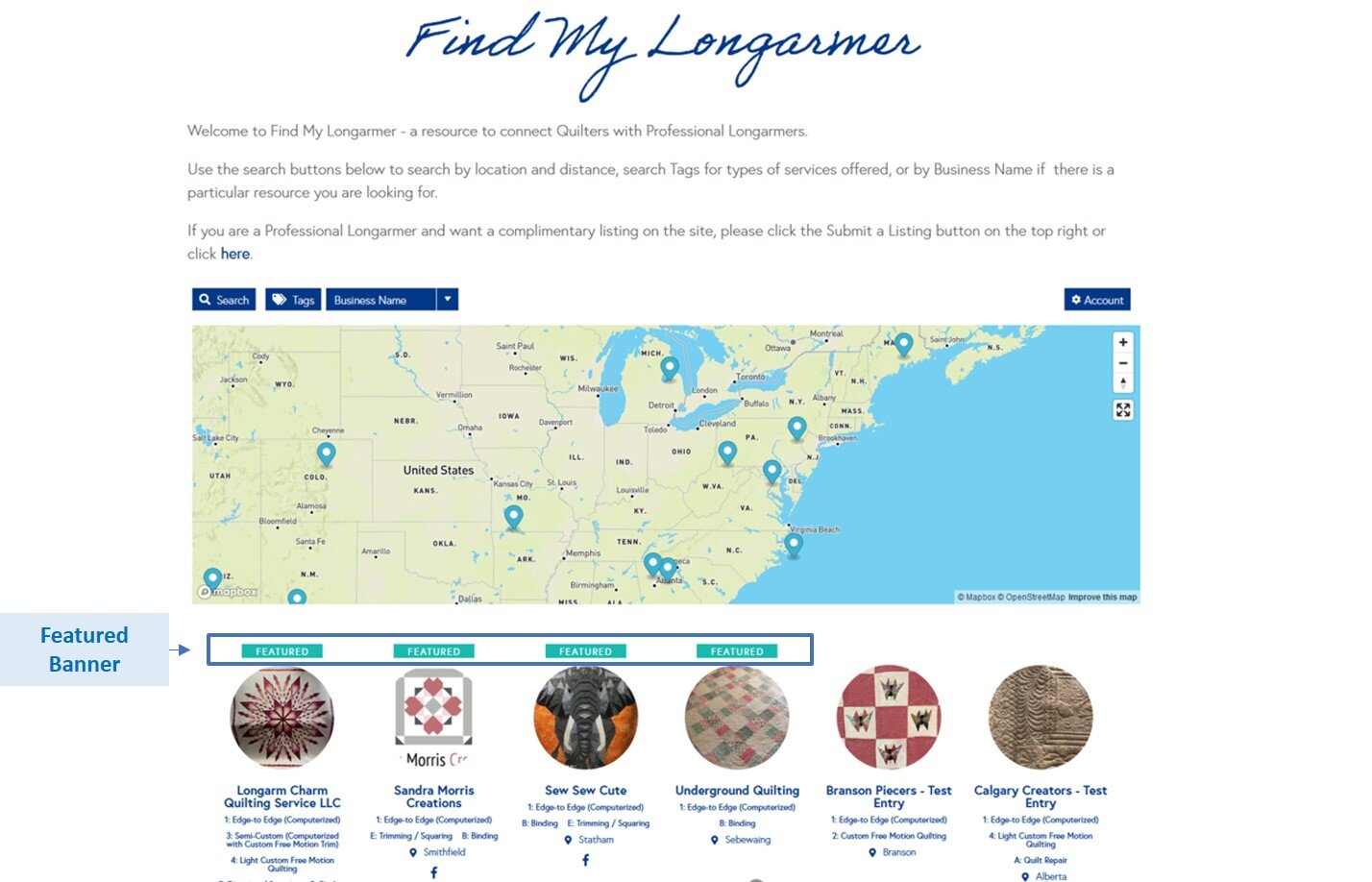This is an image of a webpage designed on a white background, devoid of any borders. At the top of the screen, in elegant navy blue script, the text "Find My Longarmer" is displayed. Below this, in slightly smaller navy blue text, a welcome message reads: "Welcome to Find My Longarmer - A resource to connect quilters with professional long armers. Use the search buttons below to search by location and distance, search tags for types of services offered, or by business name if there is a particular resource you are looking for. If you are a professional long armer and want a complimentary listing on the site, please click the 'Submit a Listing' button on the top right or click here," with the word "here" emphasized in bold.

Beneath this text, the image features a map focusing on the eastern half of the United States, encompassing roughly 50-60% of the area. The map is dotted with numerous light blue pins, marking various locations. Additionally, prominent geographical features including part of the Atlantic Ocean and the Great Lakes are visible on the map.